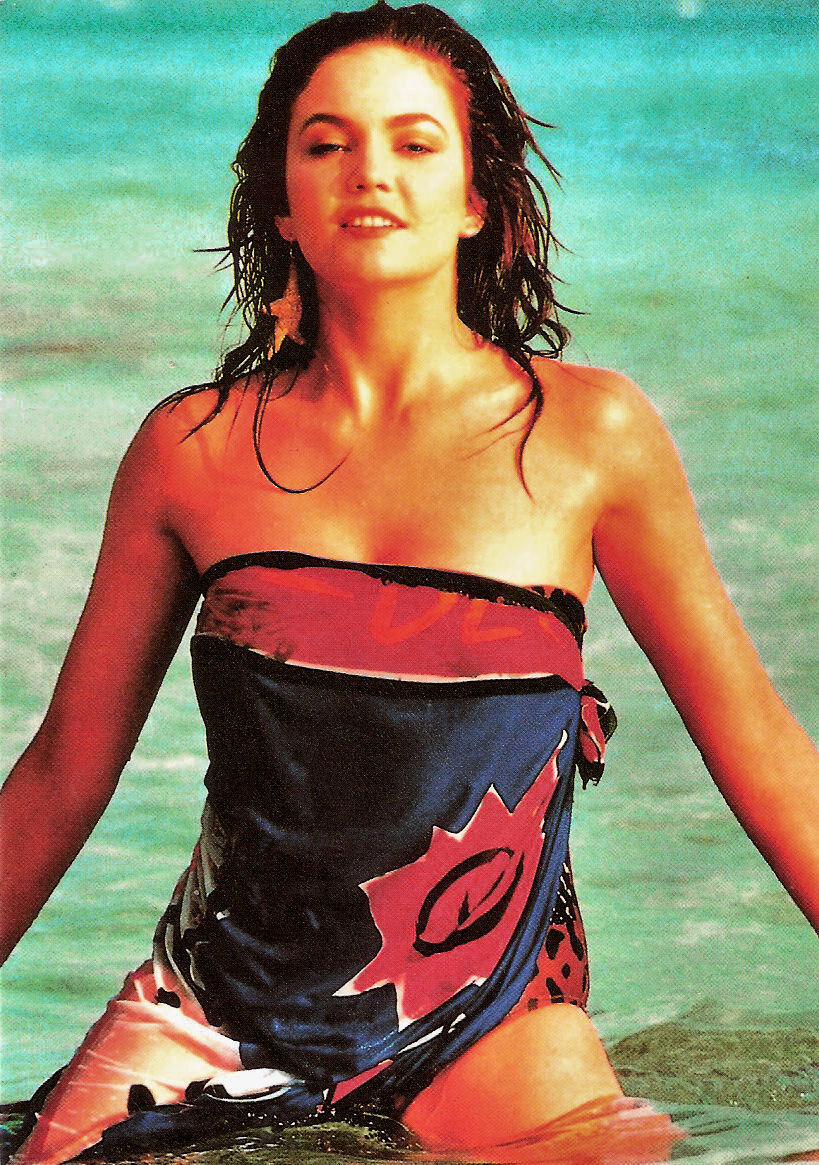In this image, we see a woman, possibly a model or actress, immersed in an expansive body of water that appears to be either a beach or pool. The backdrop of the scene showcases light blue to greenish-white water that darkens towards the edges. The woman, with her long brown hair soaked and cascading past her shoulders, is smiling gently at the camera. She is adorned with starfish-shaped earrings on her right ear, adding a touch of marine charm to her look. 

Her attire consists of a strapless dress that features a mix of pink, red, and blue hues. The dress is partially transparent towards the bottom, and it has a distinct red stripe circling her breast area. Her arms are outstretched, and she seems to be seated on something submerged in the water, with her legs partly immersed. Overall, the image captures a serene and lightly playful moment as she relishes the water's embrace.